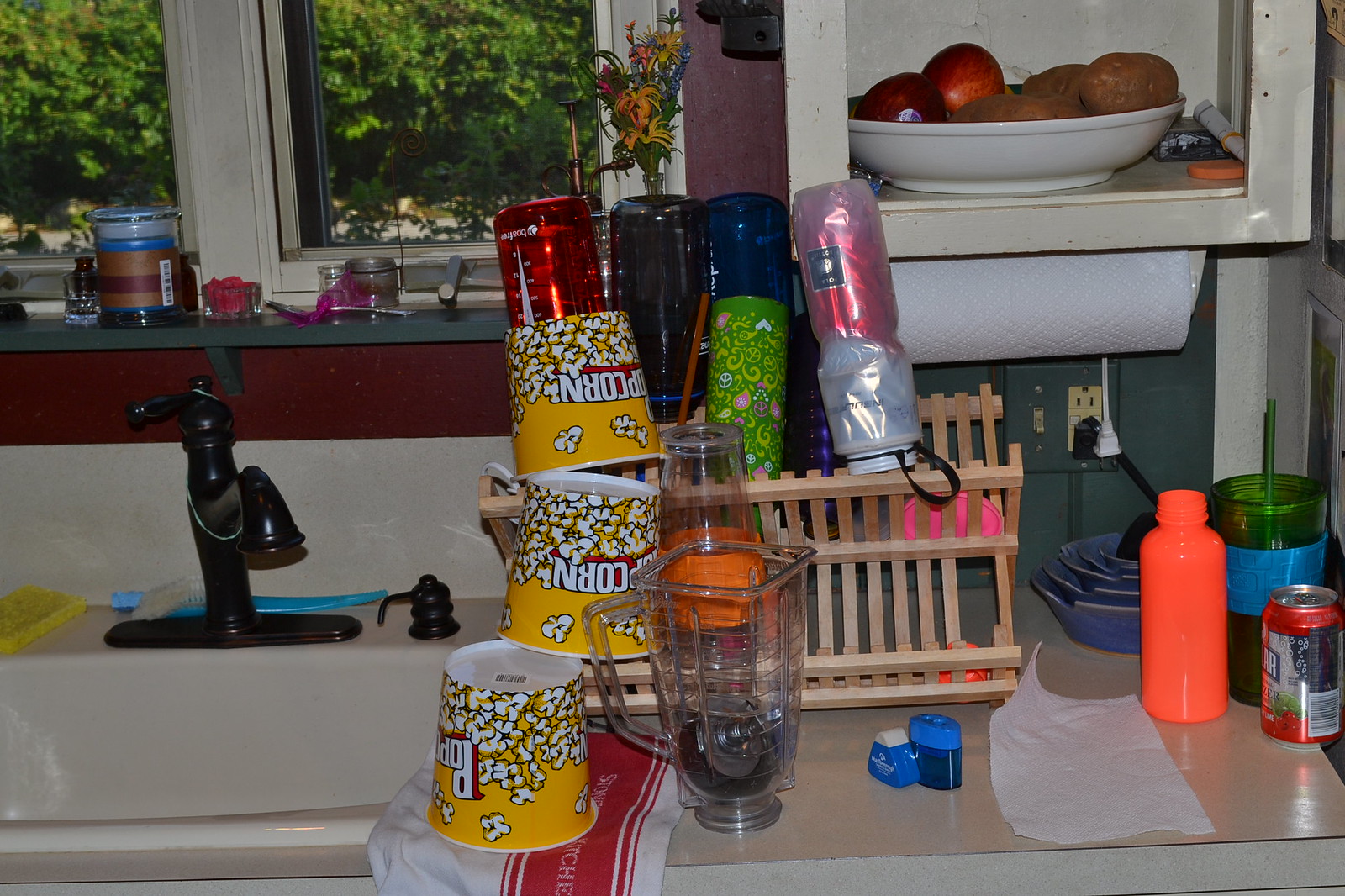On the black-faceted sink countertop, a wooden dish rack is neatly arranged, holding an assortment of bottles, cups, and recently washed popcorn buckets that are drying. Above the sink, a window offers a view of a lush green tree with vibrant leaves, while a colorful flower adorns the windowsill. To the side of the window, a white cabinet stands with a white plate on top, showcasing a collection of red apples and kiwis. Additional items on the countertop include a can of juice, an orange bottle, and a stack of blue plates.